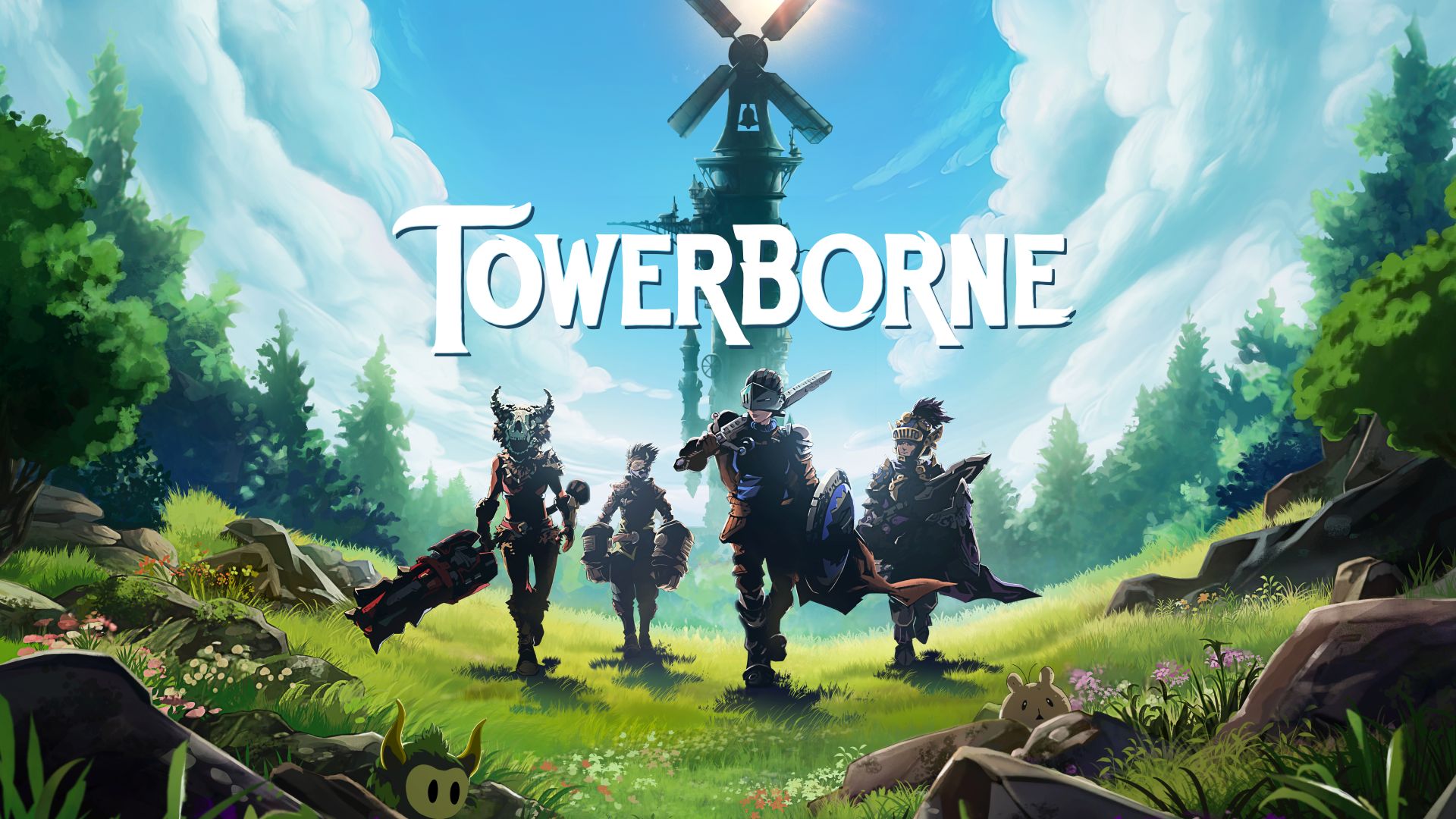The animated promotional image for the video game Towerborn (spelled T-O-W-E-R-B-O-R-N-E) features a detailed, vibrant scene. Dominating the center of the image, the title "Towerborn" is displayed in bold white text with a slight black drop shadow, seamlessly integrated into the upper third of the visual. Sitting amidst a lush, forested terrain, the narrative centers around a prominent windmill-topped tower, its silhouette set against a bright blue sky with swirling clouds that give the impression of the eye of a storm. The sun partially peeks through from behind, casting the scene in a dynamic daylight.

Marching towards the viewer through a field of green grass interspersed with rocks and small forest creatures, four characters clad in various types of medieval fantasy armor add action and life to the setting. From left to right: the first character wears a helmet bearing two outward-curving horns and wields a weapon; the second character, similarly armored, holds a massive gauntlet; the third, donning what appears to be a creature-skull helmet with horns and brandishing a huge sword; and the fourth in a traditional knight’s helmet visor is equipped with both a shield and a sword. The detailed setting and dynamic character designs together create an enticing glimpse into the adventurous world of Towerborn.